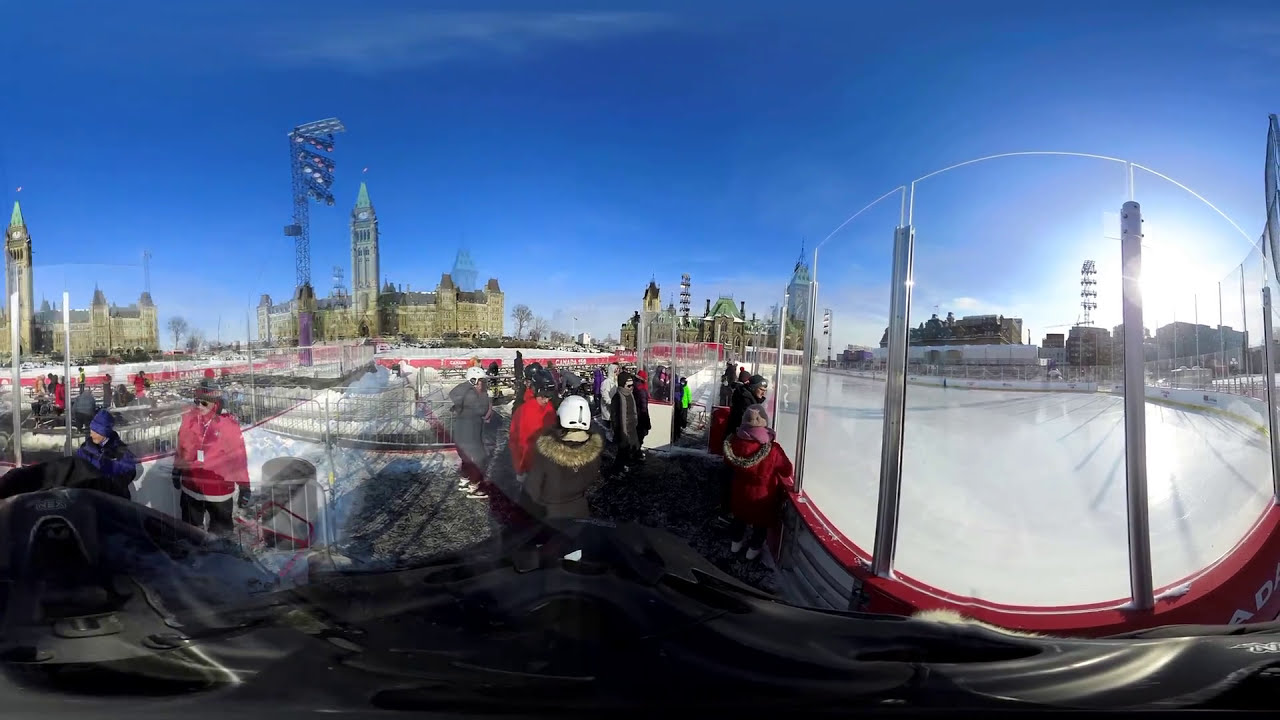This panorama image presents an outdoor ice skating rink, likely located in a Canadian setting, given the architectural similarities to notable landmarks like the Houses of Parliament. The scene is taken with a wide-angle, 360-degree perspective, resulting in some distortion. Dominating the background is a tall clock tower and an old-style building, adding a historic charm to the atmosphere. 

In the center of the image, a group of people dressed in winter attire, including helmets, fur-trimmed coats, and beanies, are waiting in line. On the right, the expansive ice rink is bordered by glass walls, indicating a designated area for either ice skating or hockey, though it currently stands empty. To the left, there is metal fencing and patches of snow on the ground, enveloping the scene in a typical winter setting. The bright blue sky with sparse, wispy clouds overhead encapsulates the daylight ambiance, lending a clear and vivid quality to the photograph. Overall, the image captures a bustling yet serene winter scene illuminated by natural sunlight.